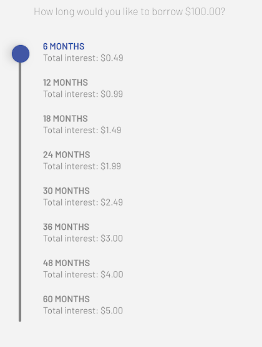This vertical image is a low-resolution screenshot showcasing a portion of a questionnaire with visible pixelation upon zooming. The background is a light gray, and at the very top, there's a medium gray text that reads, "How long would you like to borrow $100.00?" Below this question, a series of options are displayed, each representing different loan durations and their corresponding total interest.

A vertical slider is positioned on the left side, currently pushed to the top of a navy blue vertical line. The slider itself is marked by a dark navy blue circle, indicating the selection of the topmost option. This highlighted option is "6 months," written in blue font, accompanied by the total interest of "$0.49."

The subsequent options listed below include:

- 12 months, total interest $0.99
- 18 months, total interest $1.49
- 24 months, total interest $1.99
- 30 months, total interest $2.49
- 36 months, total interest $3.00
- 48 months, total interest $4.00
- 60 months, total interest $5.00

Each option details a longer borrowing period with a progressively higher total interest.